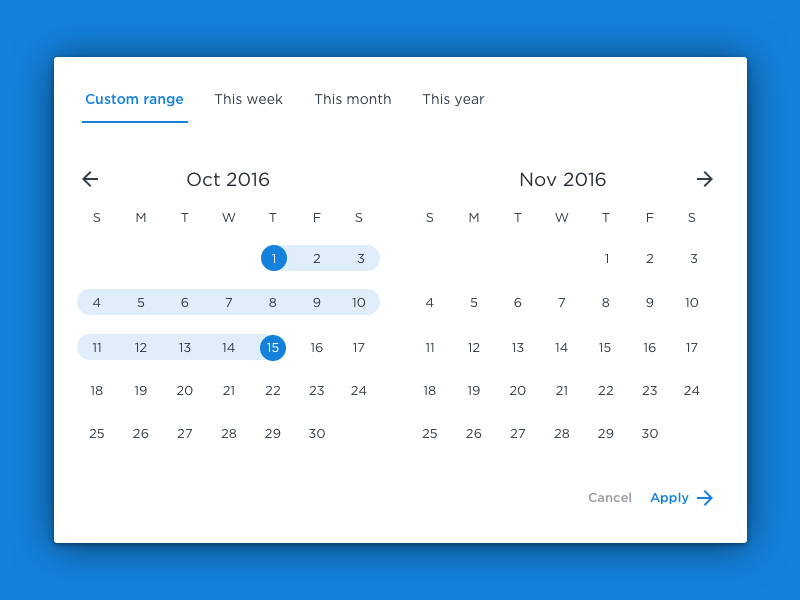The image is a screenshot from a computer displaying two calendar pages against a royal blue background. The main focus is a white rectangle positioned in front of the blue backdrop, containing calendar pages. On the left side, the calendar shows October 2016, while the right side displays November 2016. At the top of this white rectangle, there is an option labeled "Custom Range" in blue font and underlined. To the right of it, in black font, are the labels "This Week," "This Month," and "This Year."

For the October 2016 calendar, there is a left-pointing arrow located at the top left corner, indicating the option to navigate to September. Likewise, an arrow next to November 2016 points to the right, allowing navigation to December. Within the October calendar, the dates from the 1st to the 15th are highlighted, with both the 1st and the 15th featuring blue circles around them.